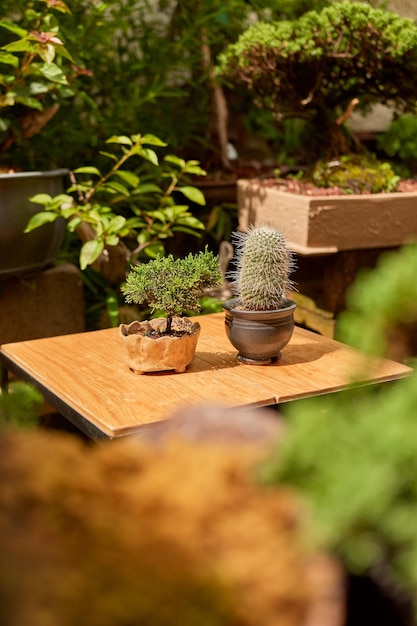In the garden area outside someone's house, we see a well-maintained and thoughtfully designed arrangement of various potted plants. Dominating the scene in the middle is a small, light brown, square wooden table. Atop this table on the left side sits a miniature tree that resembles a bonsai, planted in an earthy round pot with distinct ridges on the top. The tree has a tiny dark trunk supporting a large, lush bush of green foliage. On the right of the table, there is a shiny gray round pot containing a single, robust cactus. Throughout the background, a variety of other green and brown plants are visible, contributing to the warm, garden-like atmosphere. The image exudes a soft, warm glow, and the foreground is softly blurred, with beige and green hues blending gently out of focus. This setting showcases an array of plants, adding a serene and organic touch to the outdoor space.